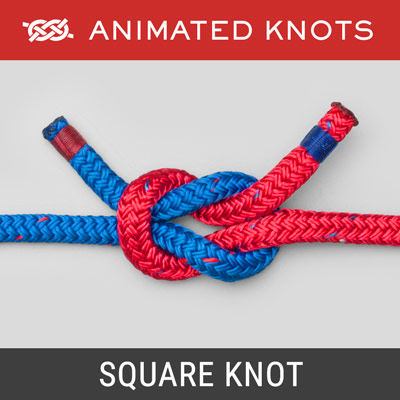This square image serves as an instructional infographic on tying a square knot. Dominating the top of the image is a red banner featuring white text that reads "Animated Knots," accompanied by a simple knot illustration on the left. The center of the image displays a detailed visual of a square knot, where a blue rope and a red rope interweave and loop together tightly, with the blue rope winding under and over the red rope, and vice versa. The finely wrapped ends of each rope feature alternating colors - blue rope with a red wrap, and red rope with a blue wrap. At the bottom, a dark gray banner in white text labels the knot as a "Square Knot." The main colors of the graphic are white, red, blue, and black, highlighting the knot as the central focus.